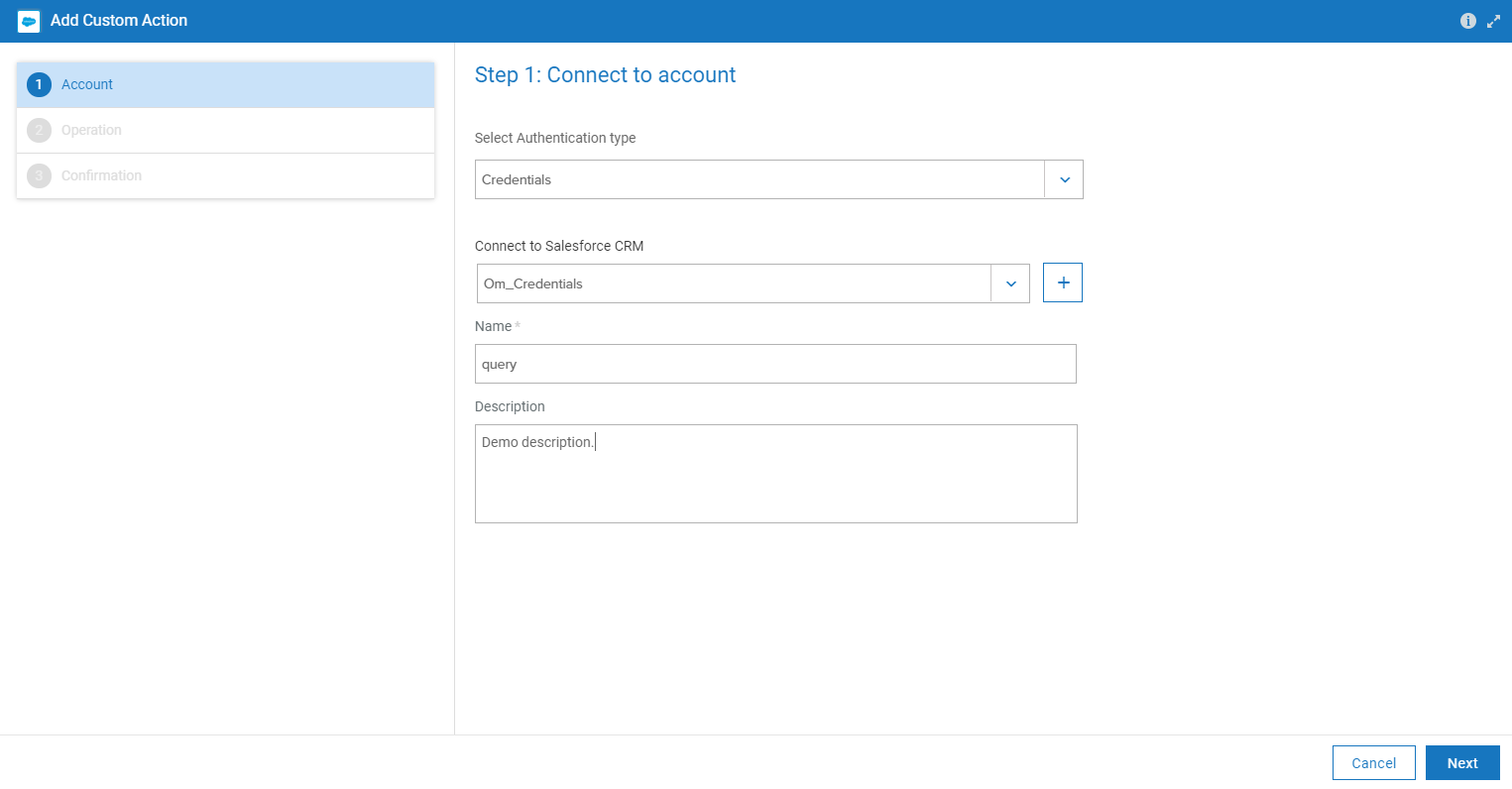This image appears to depict a series of screenshots from a website interface, possibly related to a configuration or setup process. 

At the top of the image, there's a dark blue horizontal bar. On the left side of this bar, there's a white square icon containing a blue cloud. To its right, in light blue text, it says "Add Custom Action." On the far right, there's a gray circle featuring an eye icon within it, colored blue. Adjacent to this, there are two gray arrows, one pointing up and the other pointing down.

Below this top bar, there's a small menu containing three headings. The first heading is highlighted in blue and includes a blue circle with a white number one inside it, labeled "Account" in blue. The second heading features a gray circle with a gray number two inside it, labeled "Operation" in gray. The third heading shows another gray circle with a gray number three inside it, labeled "Confirmation" in gray.

In the middle of the page, a blue text indicates "Step 1: Connect to Account." Under this instruction, in black text, it says "Select Authentication Type," followed by a drop-down menu. The drop-down menu displays "Credentials," with downward blue arrows on both the left and right sides. Below this, another title in blue text reads "Connect to Salesforce CRM." Directly underneath, there's another menu box labeled "OM_Credentials," accompanied by downward-facing arrows on either side. To the right of this menu box, there is a blue square with a white interior and a blue plus sign inside it.

Further down on the left, gray text indicates "Name," and within a horizontal gray box, it says "Query." Underneath, it reads "Description," followed by another gray outlined horizontal box with a white interior that says "Demo Description" in gray text.

In the bottom right corner of the screen, there are two buttons. The "Cancel" button is white with blue letters, and to its right, the "Next" button is dark blue with white letters.